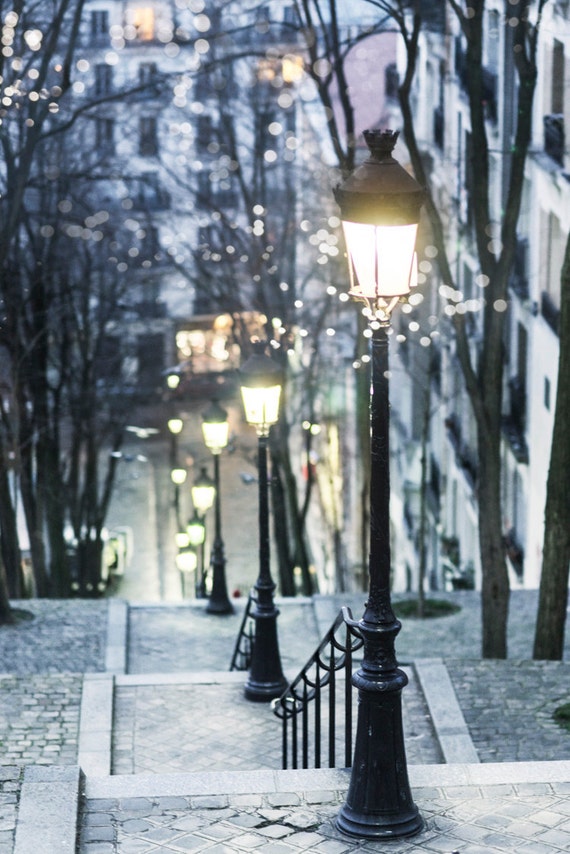This photograph captures a nighttime scene of a broad brick stairway descending a hillside in a city or town. The stairway, composed of irregularly patterned bricks, is bordered on both sides by leafless trees, suggesting it is winter. Black wrought iron railings run down the middle of the steps, which are punctuated by a series of at least ten vintage-style black lampposts. The lampposts, each crowned with ornate tops, cast bright white light that illuminates the gently falling snowflakes around them, though the ground remains clear of snow. In the blurry background, several buildings, possibly five stories tall, frame the scene, adding to the urban ambiance.